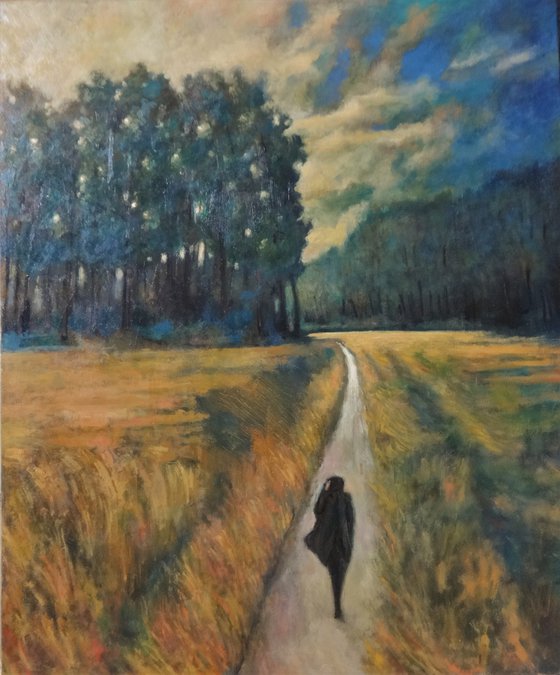The detailed painting captures a lone silhouette of a woman walking down a long, paved pathway that stretches into the distance, eventually curving and disappearing behind a grove of tall, thin trees. The pathway is flanked by tall, brown and yellow grass which create a prairie-like setting on either side. The sky overhead is a mix of vibrant blue with scattered, white and brown-tinged clouds, adding a dynamic feel to the scene. The artwork employs a detailed, oil pastel technique, using numerous strokes to bring texture and depth to the natural surroundings.